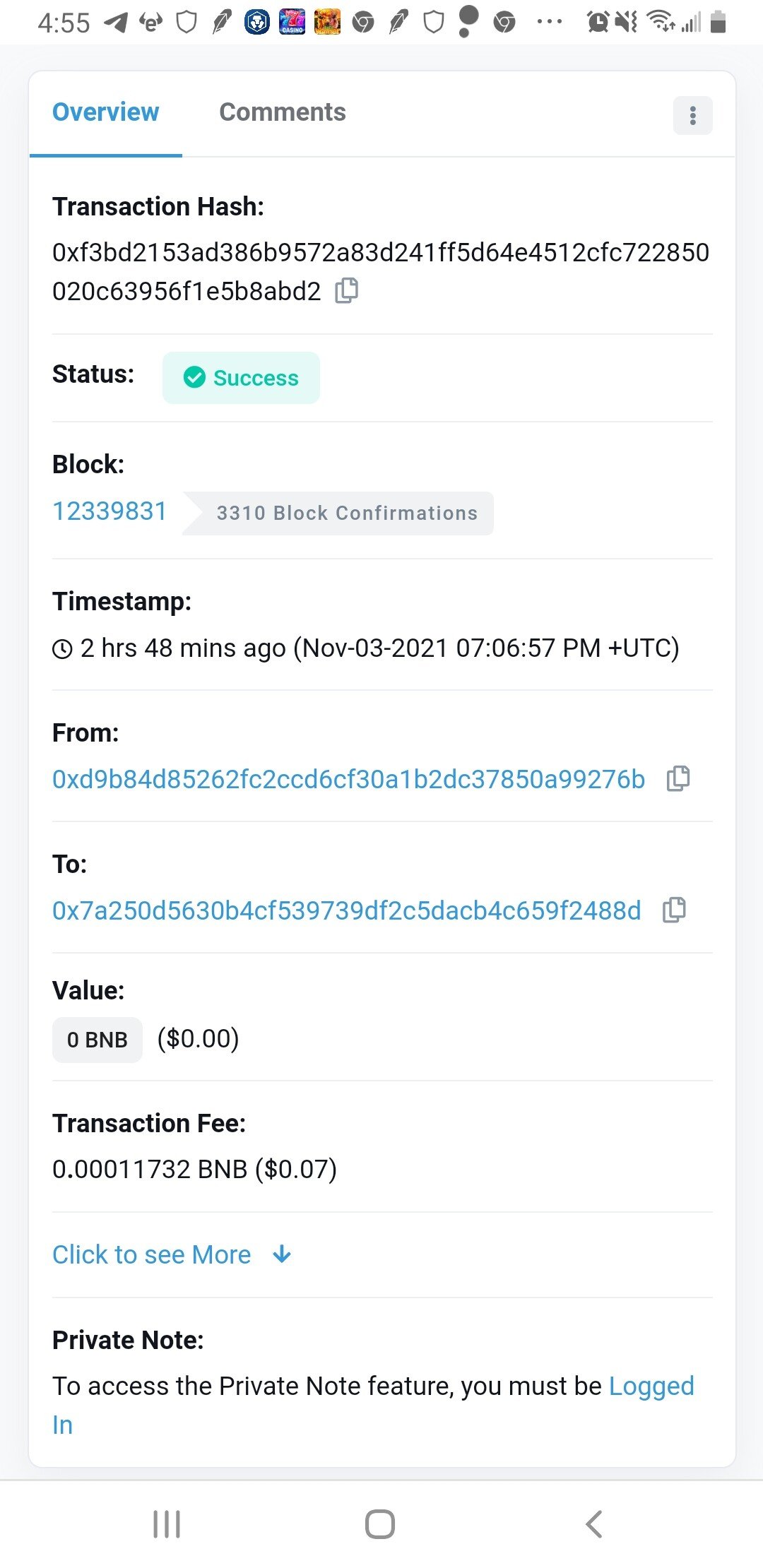The image is a screenshot of a cell phone displaying the "Overview" section of an app interface. The "Overview" tab is highlighted in blue with a blue underline indicating it is the active section. Under the "Overview" heading, there is a "Transaction Hash" with a line of alphanumeric text partially visible. At the end of this line, there is a copy symbol, allowing the user to copy the hash to their clipboard.

Below the "Transaction Hash," there is a "Status" section that indicates the status of the transaction as "Success." The next section, labeled "Block," displays a block number "333110," accompanied by a gray bar and confirmation status of "1 block confirmation." The "Time Stamp" section below provides a timestamp indicating that the transaction occurred "2 hours and 48 minutes ago on November 3rd, 2021, at 7:06:07 PM."

Further down, there is an "From" section, followed by a "To" section, and finally, a "Value" section, although specific details for these sections are not provided in the visible portion of the screenshot. The app interface is clean and organized, presenting all relevant transaction details clearly for the user.